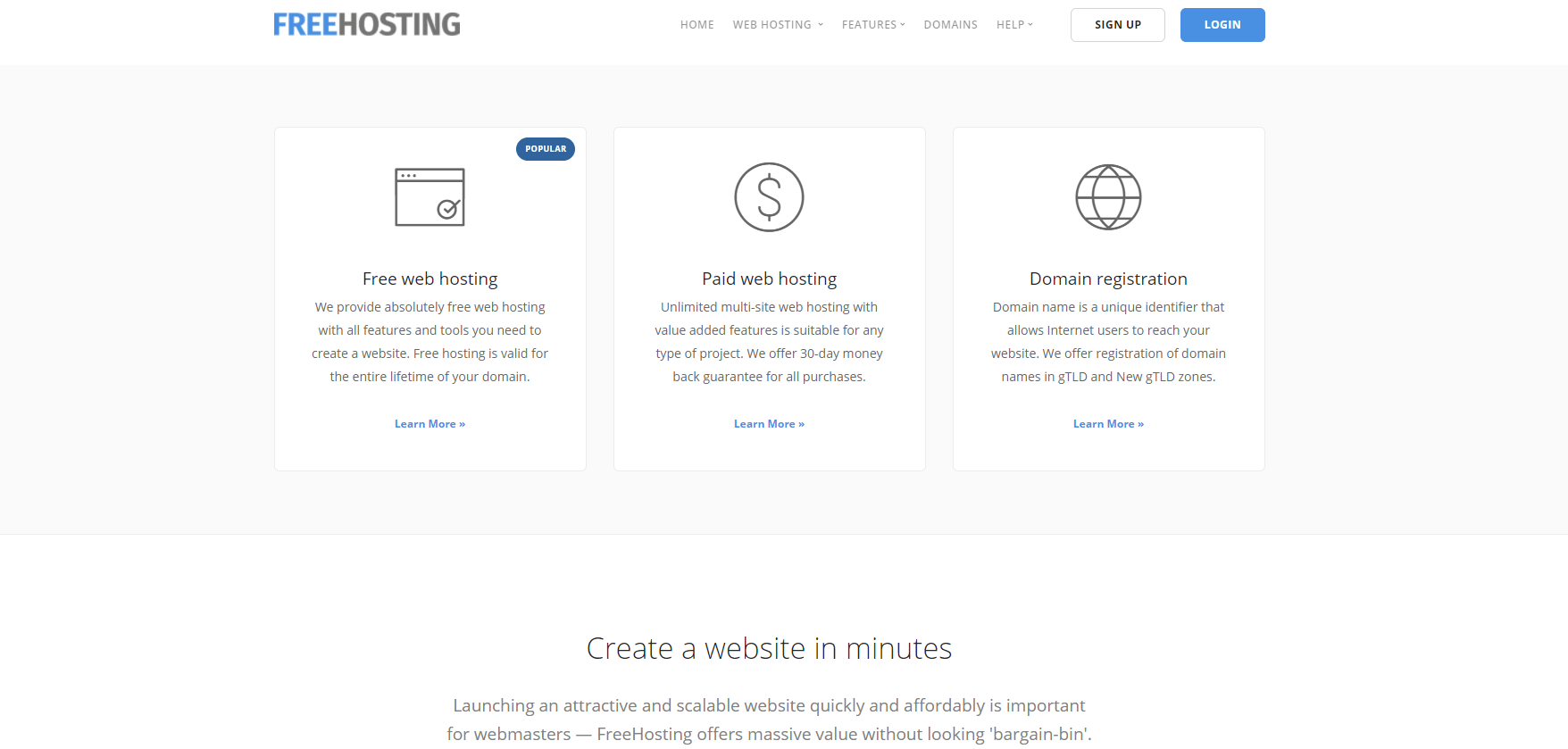**Screenshot of Web Hosting Service Web Page:**

The upper left corner of the page prominently features "FREE HOSTING" in capital letters, with "FREE" in a distinctive blue color and "HOSTING" in black. Directly to the right of this heading, there are navigation tabs for "HOME," "WEB HOSTING," "FEATURES," "DOMAINS," and "HELP," all in capital letters.

Further to the right, a white box with black text reads "SIGN UP," while a blue box with white text says "LOG IN." 

Beneath the navigation bar is a light gray banner, housing three key offerings in white boxes. 

- **First Box (Left):** 
  - Upper right corner: a blue circle with white text labeled "POPULAR."
  - Image: A depiction of a webpage with a circle containing a check mark.
  - Text: "Free Web Hosting. We provide absolutely free web hosting with all features and tools you need to create a website. Free hosting is valid for the entire lifetime of your domain." The words "Learn more" are in blue.

- **Second Box (Middle):** 
  - Image: A circle with a dollar sign.
  - Text: "Paid Web Hosting. Unlimited multi-site web hosting with value-added features is suitable for any type of project. We offer a 30-day money-back guarantee for all purchases." The words "Learn more" are in blue.

- **Third Box (Right):** 
  - Image: A picture of a globe.
  - Text: "Domain Registration. A domain name is a unique identifier that allows internet users to reach your website. We offer registration of domain names in various gTLD and new gTLD zones." The words "Learn more" are in blue.

At the bottom of the banner, a concluding statement reads, "Create a website in minutes. Launching an attractive and scalable website quickly and affordably is important for webmasters. Free hosting offers massive value without looking bargain bin."